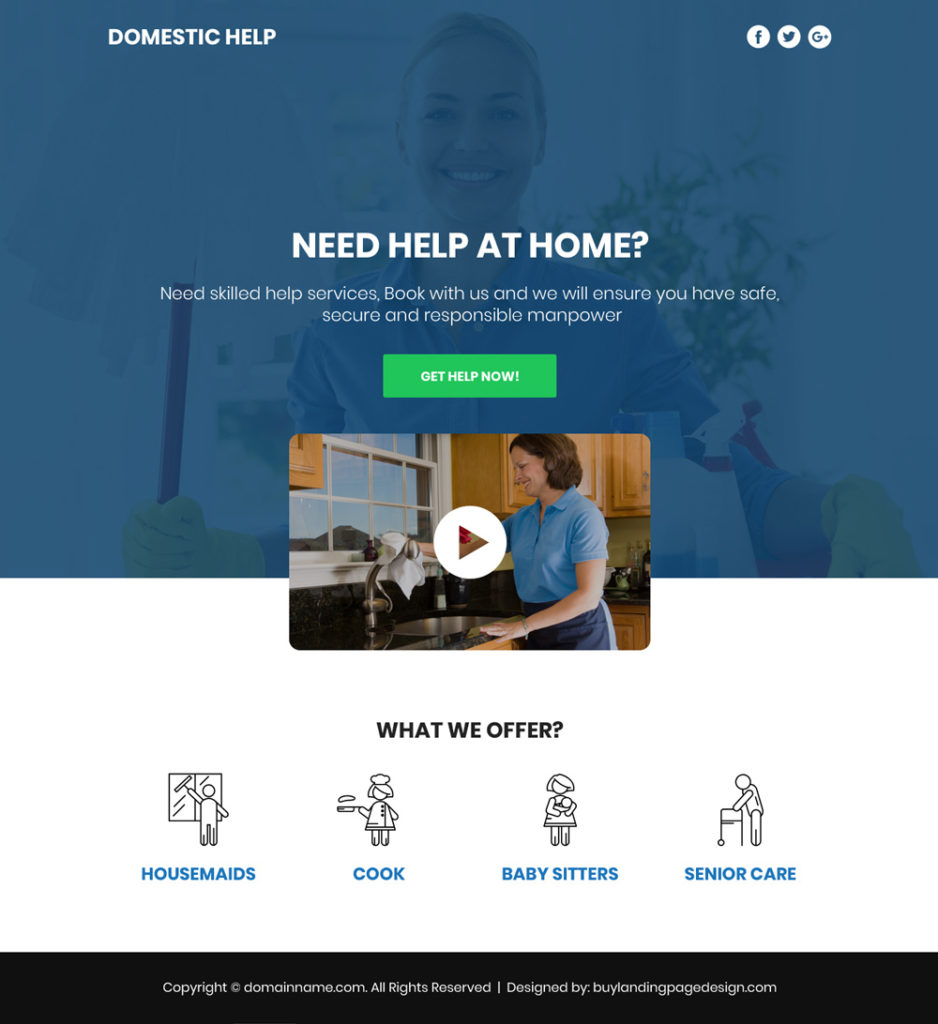This detailed caption describes the elements and design of a mock-up landing page template, likely for sale, that focuses on domestic help services:

The top left corner features the title "Domestic Help," while the top right corner displays icons for Facebook, Twitter, and Google Plus. Beneath the header is an image of a Caucasian woman, who appears to be a maid, positioned in front of cleaning supplies. She has blonde hair, a blue shirt with rolled-up sleeves, and is slightly obscured by a 70% opaque blue overlay, allowing the text to remain prominent. Behind her, a window with a plant can be partially seen.

In large white text, the page prominently states: "Need help at home." Below this, smaller text reads: "Need skilled help services? Book with us and we'll ensure you have safe, secure, and responsible manpower." A green button underneath, with white text, encourages action with the message: "Get Help Now!"

Centered on the page is a video thumbnail featuring a woman smiling as she cleans a sink, set within a kitchen with a granite countertop. The video thumbnail includes a play button symbol—a translucent triangle over a white circle.

Further down, four icons represent different services: housemaids, cooks, babysitters, and senior care, each accompanied by blue text.

The footer of the page displays the copyright statement: "© [Domain Name], All Rights Reserved," and credits the design to "landingpage.design.com."